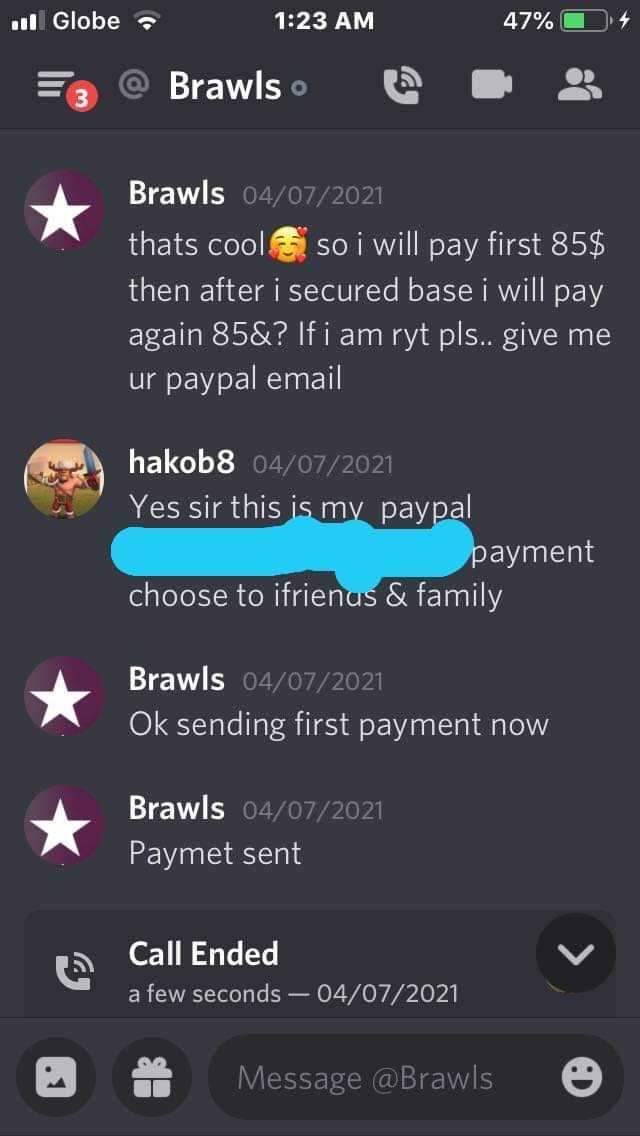This detailed screenshot from a messenger app on a mobile phone shows a conversation between two users, Brawls and Hakob 8. Across the top of the display, you can see standard phone indicators such as the time (1:23 a.m.), battery percentage (47%, charging), Wi-Fi signal, and reception bars, confirming it as a mobile screenshot. The interface hints it might be Discord, featuring icons for a telephone, video call, and contacts next to the chat label "Brawls." 

The conversation starts with Brawls, highlighted by a star, sending a detailed message: "That's cool 😊. So I will pay first $85 then I secure the base. After I secure the base, I will pay again $85, and if I am our YT PLS...give me your PayPal email." Hakob 8 promptly responds with his PayPal details and specifies, "Yes, sir. This is my PayPal," although some parts are obscured. He advises to select "friends and family" for the payment type. Brawls then confirms with, "Okay, sending first payment now," followed by "payment sent." The conversation concludes with "call ended," indicating the end of their interaction.